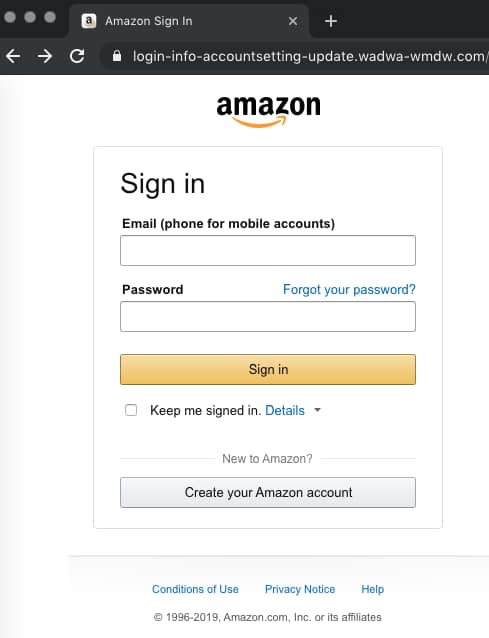The image is a cropped screenshot of the Amazon sign-in page captured within a browser tab. At the top, the browser interface is set to a black theme, featuring three gray circles on the far left. Next to these circles, there's a darker gray tab displaying the Amazon favicon, a stylized "A" with a yellow arrow underneath. The tab is labeled "Amazon sign-in," followed by a small "X" to close the tab. To the right, there is a plus sign for opening a new tab.

Directly below the tabs, the browser UI includes navigation buttons: a left-arrow for 'back', a right-arrow for 'forward', a reload button, and an almost black URL search bar with a white padlock icon, indicating a secure connection. The URL partially visible reads "login-info-accountsending-update.wmdw.com/..." where the text abruptly ends due to the cropped nature of the screenshot.

Focusing on the main content within the browser, the top center features the Amazon logo with its signature yellow underline. Below that, a thin gray-lined rectangle encompasses the sign-in form. Prominently displayed in large, black, sentence-cased letters is "Sign-In." Underneath, in smaller bold text, it reads "Email (phone for mobile accounts)" with an empty input field below it.

Further down, the word "Password" is displayed in bold, black letters. Adjacent to it, there’s a blue "Forgot your password?" link. Another empty input field appears below this text. The centerpiece of the form is the "Sign-In" button, designed with a yellow to darker yellow gradient, and black text in its center.

Below the sign-in button is an unchecked checkbox labeled "Keep me signed in" beside a blue "Details" link with a dropdown menu. At the very bottom, it reads "New to Amazon?" followed by a button to "Create your Amazon account."

The footer of the page contains links labeled "Conditions of Use," "Privacy Notice," and "Help." Lastly, a copyright notice reads "© 1996-2019, Amazon.com, Inc. or its affiliates."